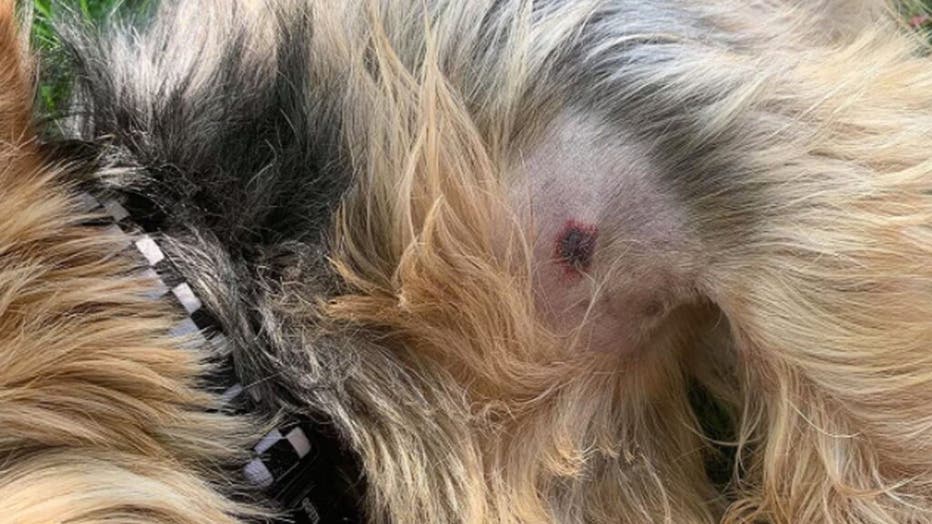The photograph is an up-close image of a dog's neck, featuring a prominent sore. The dog, possessing medium-length fur that is a mix of white, brown, and black, wears a visible black and white checkered collar. The collar has an alternating pattern of black and white squares, which is inverted along the top, forming a classic checkerboard design. The dog's fur is mostly beige with patches of black, and it has been meticulously shaved away around the wound, forming a rectangular area that showcases the sore. The sore itself is an oval shape with a dark, bloody red color, possibly indicating an infection or an injury. Positioned just below or behind the ear, the hair around this patch is brushed away to emphasize the wound. The image also captures a bit of the grass on which the dog is laying, found at the top and top right corners of the frame. The dog appears to be stationary, with no other visible injuries or disruptions in its fur.